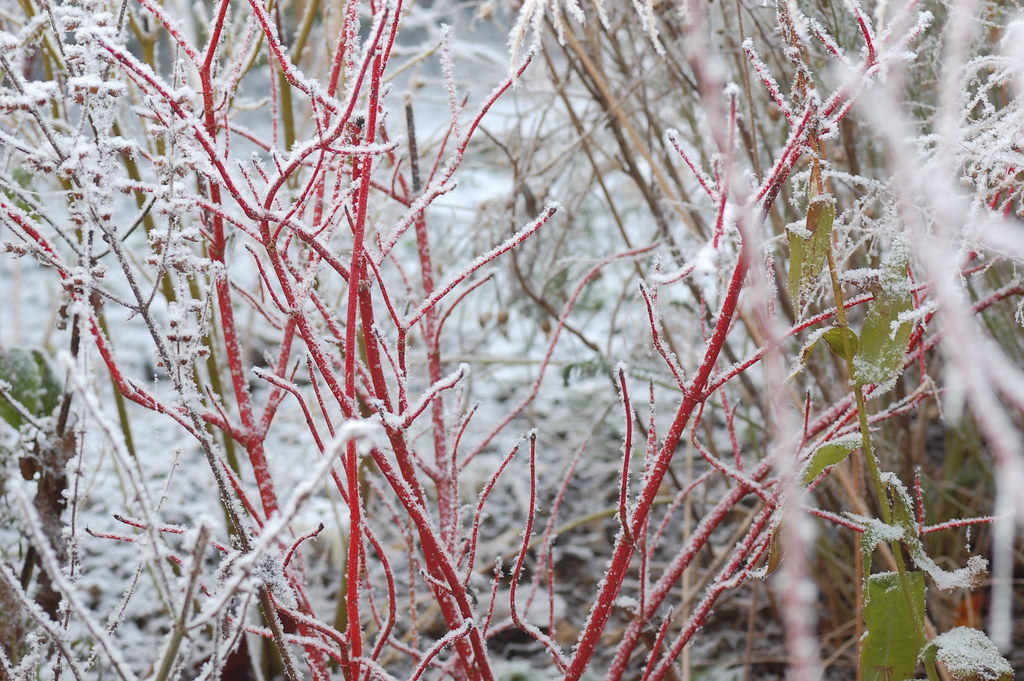The image showcases a serene forest scene, enveloped in a light dusting of fresh snow. In the foreground, the focal point is a cluster of striking red stems or branches, likely from small bushes or young trees. These vivid red stems stand out against the frosty background, a rare and captivating sight amidst the usual greenery. The left side of the image features some darker, brownish branches, while the right side displays thicker, green branches. Scattered throughout the ground are random patches of brownish branches and some leaves, all lightly covered by the thin layer of snow. The background fades into a blur of white, emphasizing the snow-covered ground and contributing to the overall tranquil atmosphere of the scene.